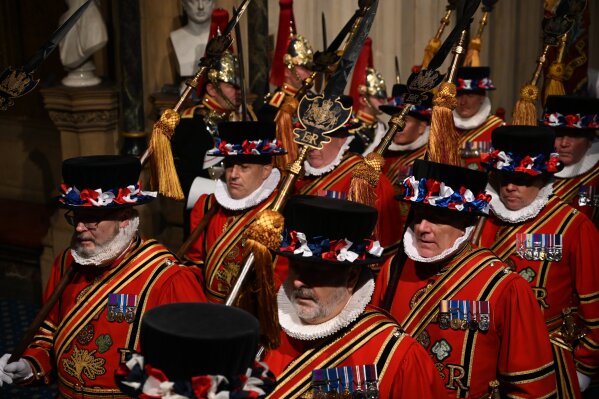This photograph captures a ceremonial display featuring the Yeoman of the Guard, also known as Beefeaters, at the UK Parliament. The image showcases about ten gentlemen adorned in elaborate red and gold uniforms with intricate black and gold stripes. They are distinguished by their large, white ruffled collars that flare out from their necks. Each wears a black top hat embellished with red, white, and blue artificial flowers encircling the band. Their chests boast an array of medals, and they carry ornamental staffs. These staffs are topped with the letters "ER" and a decorative shield design. The setting appears to be an indoor hall adorned with paintings and a bust, adding a historical ambiance to the scene. The Yeoman of the Guard are marching in unison, exuding a sense of solemnity and tradition as they partake in what seems to be a ceremonial parade or an arm salute, possibly in honor of the Queen or another significant figure.